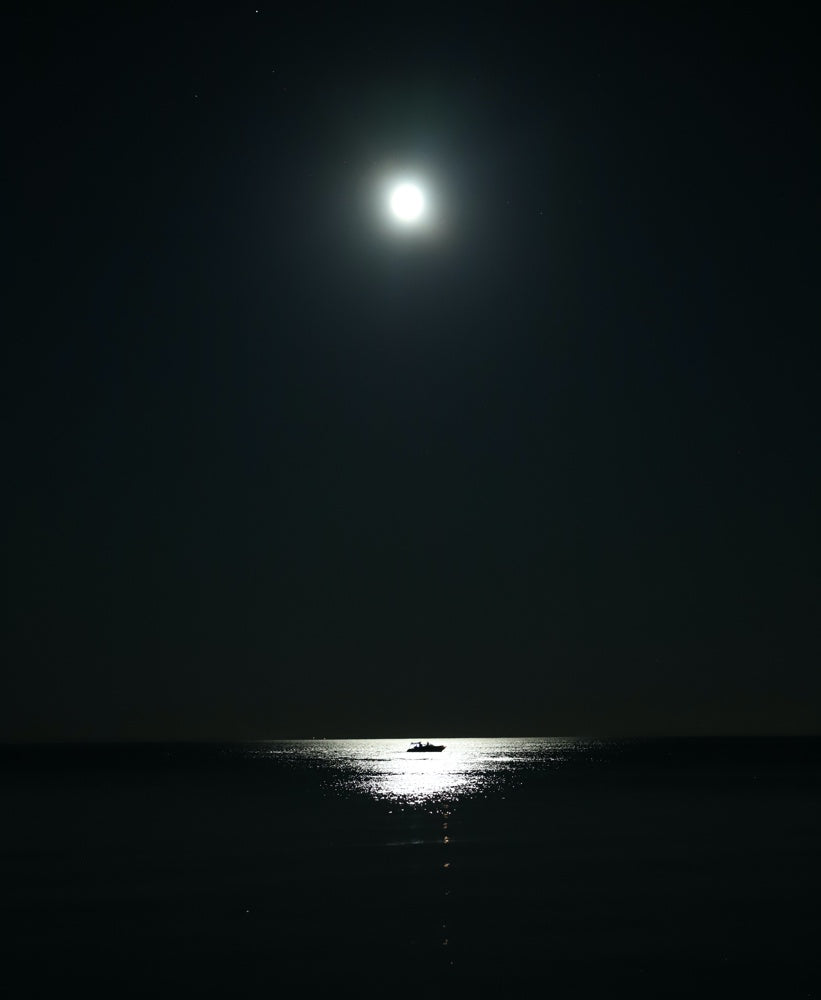This black-and-white photograph, likely taken at night, portrays a serene and solitary scene dominated by the glow of the moon in the top section. The moon's reflection creates a luminous path across the water, centrally illuminating a boat traveling from left to right. The boat is positioned right in the middle of the reflective, bright strip on the otherwise dark ocean, its silhouette stark against the shimmering light. The horizon remains unseen, emphasizing the vastness and solitude of the open water, while everything beyond the moonlit area fades into darkness, enhancing the ethereal and tranquil ambiance of the scene.